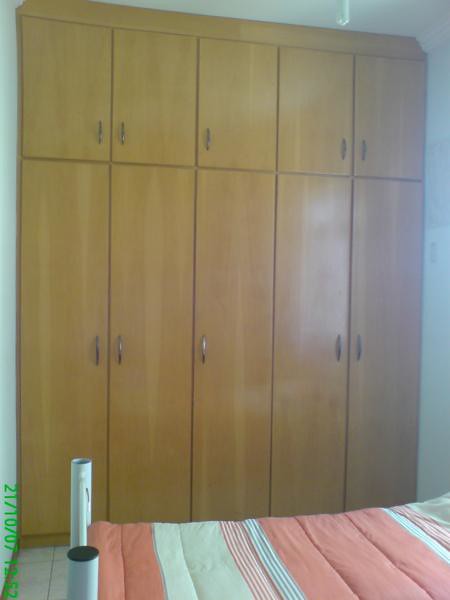The image depicts a modest bedroom, likely in a budget hotel or a dormitory in a warm country, suggested by the tiled floor and absence of carpet. The tiled floor is beige in color. The lower right corner of the image shows a basic bed with a metal frame resembling scaffolding tubes, one of which appears to have a missing plastic stopper. The bed is dressed with a pink and white striped bedsheet. Dominating the wall behind the bed is a large, light brown wooden cabinet that stretches from floor to ceiling. This cabinet is composed of five tall, slender doors on the bottom and five shorter doors on top, resembling lockers with handles for easy opening. The cabinet provides abundant storage but appears out of proportion for the small room, with its upper compartments positioned too high for practical use. Adding a touch of functional charm to the room, this cabinet accommodates locking mechanisms, although no locks are visible. In the lower left corner of the image, a green date is inscribed. The overall setting, with its simplistic design and utilitarian furniture, emphasizes functionality over luxury.